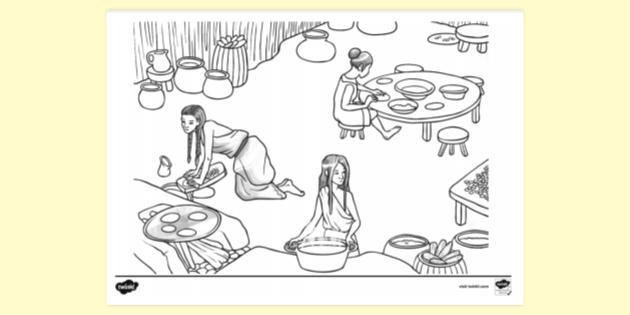The black and white drawing, sketched meticulously on a rectangular white piece of paper set against a creamy yellow background, showcases a scene of three women engaged in daily activities. On the left, a woman kneeling and washing clothes is depicted with bent knees, her hair in two braids that frame her face. In the foreground, centrally positioned, another woman stands clad in a toga, with long hair cascading down her back. She is holding a large pot releasing steam, suggesting she is cooking. Baskets holding bread and a large floor pot outline add to the scene's detail. To the right, a short, round table with various bowls is the focal point, accompanied by a woman sitting on a small stool. Her hair is neatly pulled back into a bun, and she attends to the plates and bowls on the table. In the background, there is a fence with linear patterns and numerous pots, pitchers, and a barrel adorned with flowers. This intricate representation captures the essence of a communal and industrious atmosphere, each woman deeply engrossed in her task.